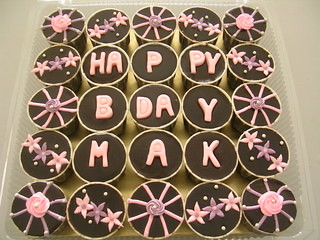In the overhead close-up image, there is a plastic case filled with 25 chocolate cupcakes arranged in a 5x5 grid, placed on a white table. The dark brown, almost black cupcakes are adorned with various intricate designs crafted from pink icing. The outer cupcakes feature ornate patterns, including rose-like swirls, clusters of two pink and one purple flower with delicate spots, and small purple flowers with black or yellow details. At the center, nine cupcakes spell out "Happy Birthday Mac" with each letter meticulously piped in pink frosting. The arrangement forms the words "H-A-P-P-Y" on the top row, "B-I-R-T-H-D-A-Y" on the middle row, and "M-A-K" on the bottom row, presumably spelling out a nickname. The image, possibly taken at a birthday party, showcases the beautiful and celebratory cupcake display.